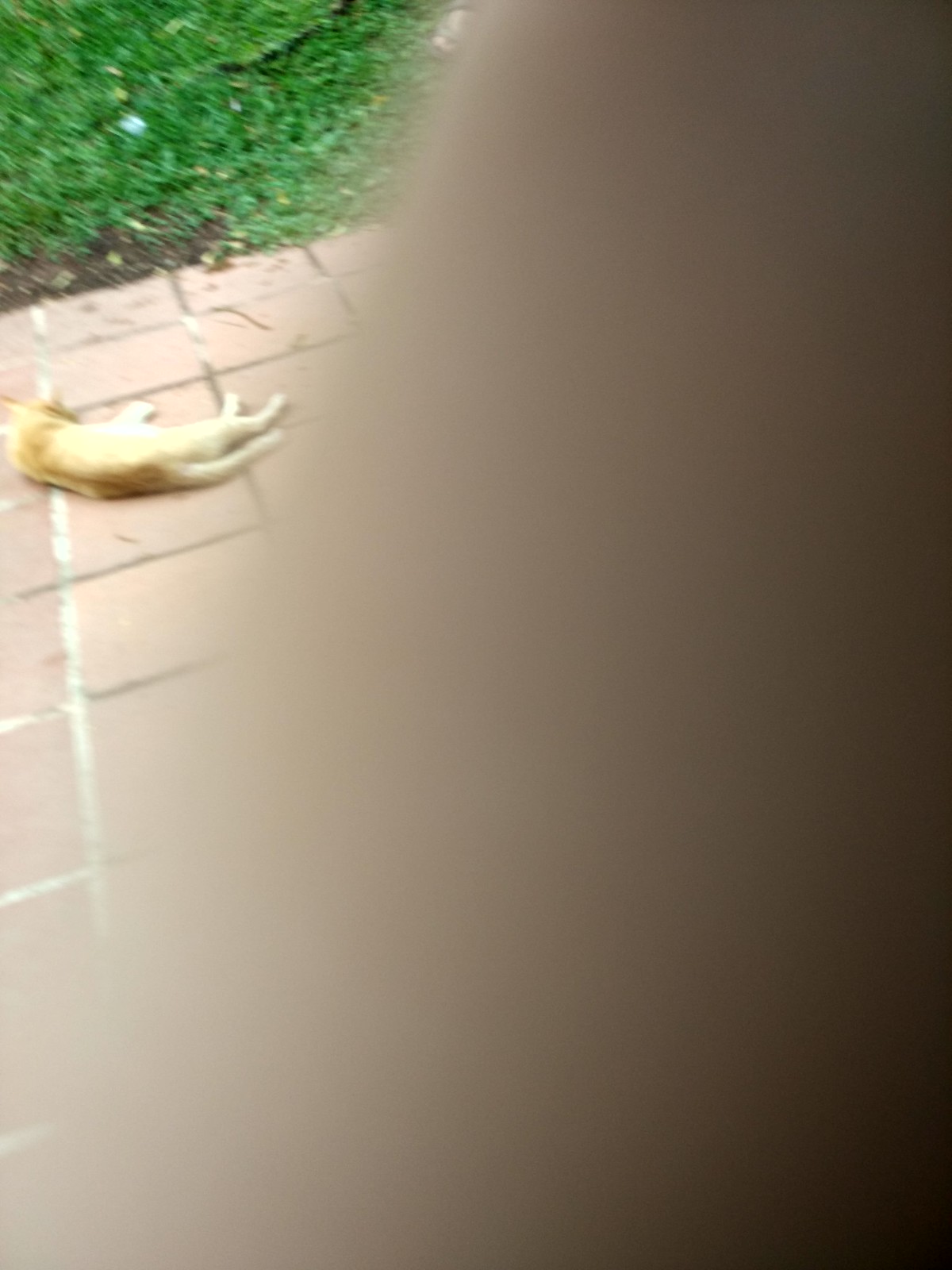This outdoor daytime photograph is largely obscured by a person's finger covering about two-thirds of the lens. The finger, which appears flesh-colored and slightly dark at the lower right, blurs the image from the lower left corner diagonally upward to nearly the middle of the top edge. Within the visible, unblurred triangular section at the upper left, the image shows a small tabby cat lying on its left side on pinkish concrete pavers. The cat's back faces the camera, with its head to the left and its tail to the right. Adjacent to the patio, a patch of green grass with a single blue flower is visible. The overall quality of the photograph is poor due to the finger obstruction and slight out-of-focus effect.